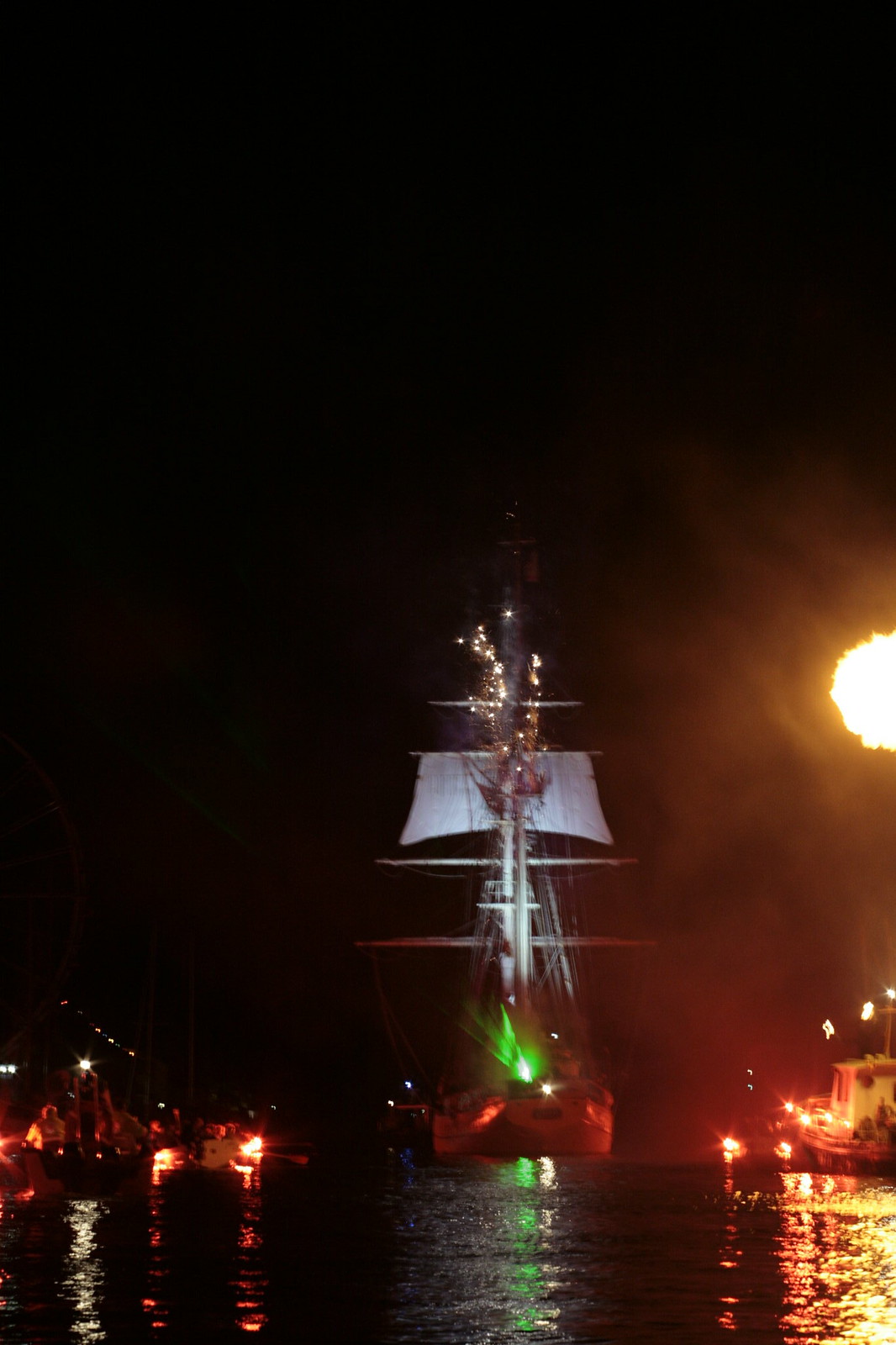In this captivating night photograph of a harbor, the focal point is a large sailing vessel, centrally positioned, that appears to be moving towards the camera. The vessel, evocative of an old pirate ship, features a prominent white elliptical mainsail and a white mast, standing out against the dark sky and serene waters. A striking green light on the ship reflects onto the calm water below, adding a mystical glow beneath the boat.

To the right side of the image, a very bright white light—possibly the moon or a strong spotlight—casts a radiant reflection onto the water. This light is so intense that it almost seems like a piece of the photograph has been bitten out, blending into the surrounding frame. In the mid-ground, both to the left and right, other boats can be vaguely seen, their yellowish-red lights twinkling and reflecting off the water's surface. Above, what appear to be fireworks or streaks of light shoot out, adding an enchanting touch to the moody nighttime scene. The water is calm, enhancing the serene and mesmerizing atmosphere of this nocturnal harbor view.